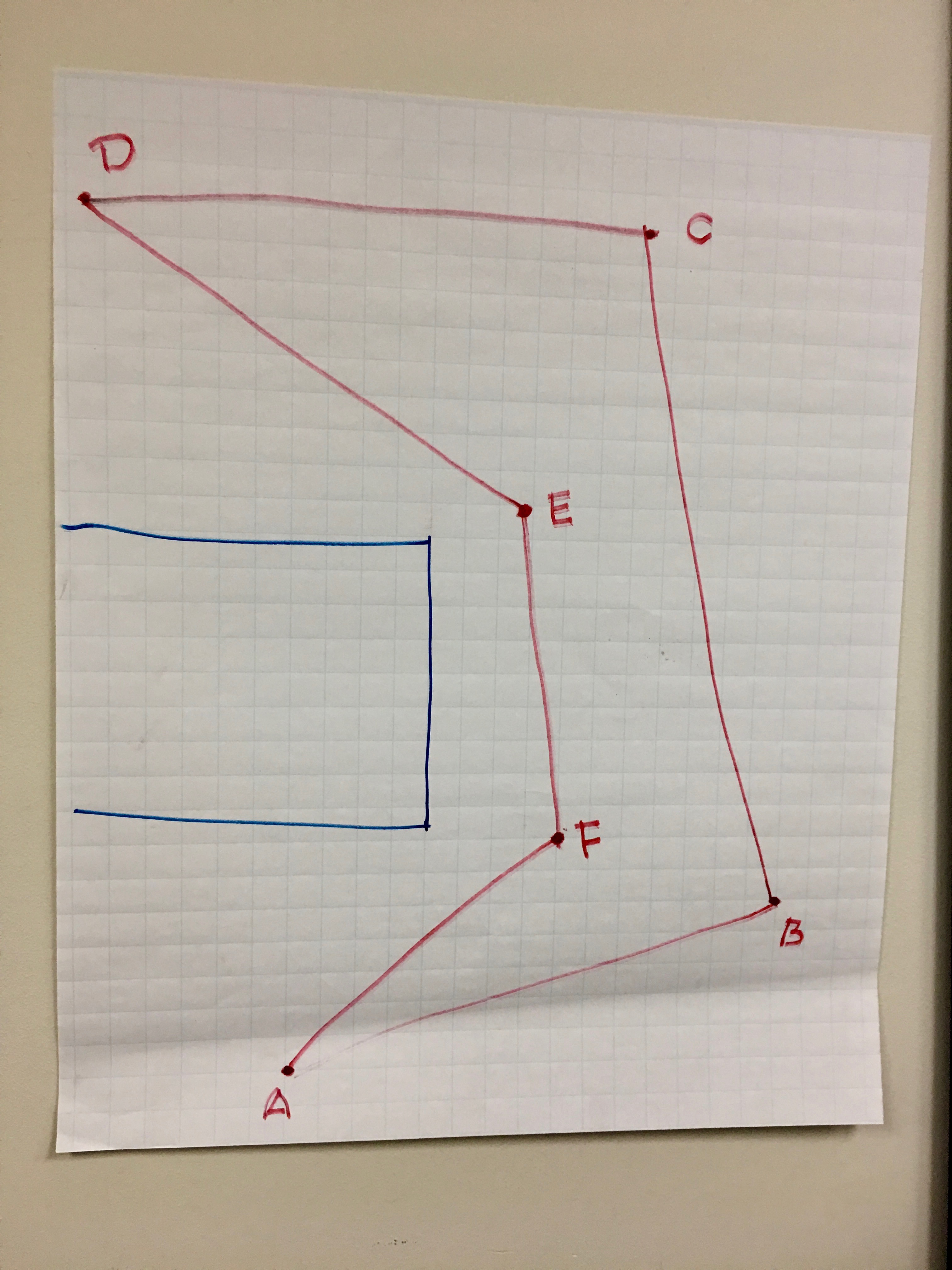The photograph portrays a detailed geometric drawing prominently displayed on a wall. The wall itself is painted in a light buff color, possibly an off-white or very light grayish-green, reminiscent of typical school or office decor. The diagram, created with markers on grid paper, is relatively large and carefully affixed to the wall. The edges of the paper curl slightly, suggesting it is mounted with tape on the backside.

Centrally positioned on the left side of the drawing is a partially visible blue rectangle. The remainder of the diagram is sketched with a red marker, though the lines appear faint, indicating the marker might be running low on ink. Below the main diagram, capital letters A through F are used as indicators, arranged as follows: A at the bottom, B to the right, C at the top, D moving to the left, E back to the right-center, and F below E.

In summary, this photograph captures a meticulously crafted geometric drawing rendered in blue and red markers on grid paper, mounted on a subdued, institutional-colored wall, with indicator letters A through F providing reference points.